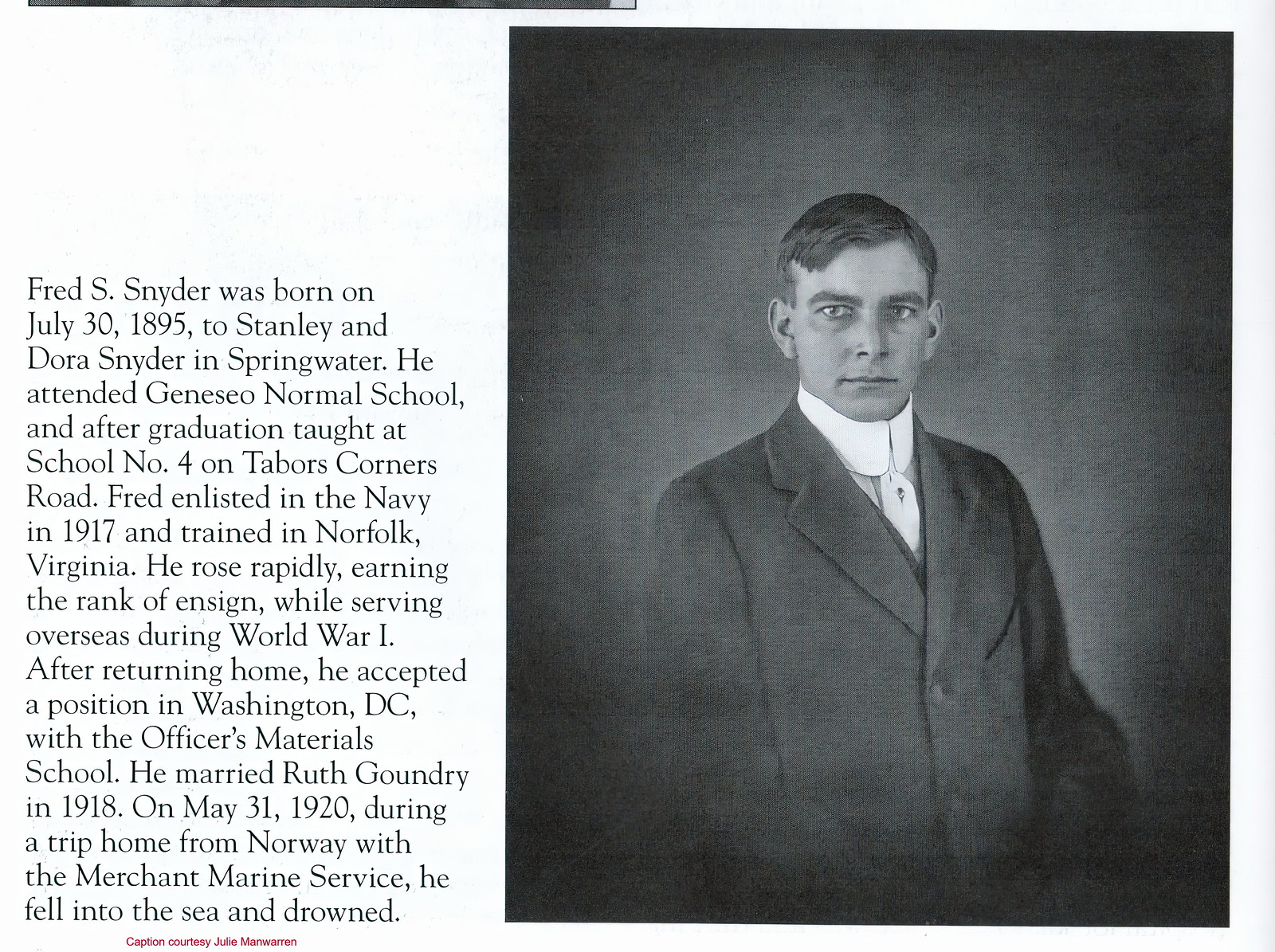This black and white image features a column of text on the left and a waist-up portrait of a man on the right. The man has short, dark hair, piercing eyes, and a wide, thin-lipped mouth. He is dressed in a dark suit, a white collared shirt, and a tie. The text beside him reads: "Fred S. Snyder was born on July 30, 1895, to Stanley and Dora Snyder in Springwater. He attended Geneseo Normal School and, after graduation, taught at School No. 4 on Tabor's Corners Road. Fred enlisted in the Navy in 1917 and trained in Norfolk, Virginia. He rose rapidly, earning the rank of Ensign while serving overseas during World War I. After returning home, he accepted a position in Washington, D.C. with the Officers' Materials School. He married Ruth Goundry in 1918. On May 31, 1920, during a trip home from Norway with the Merchant Marine Service, he fell into the sea and drowned."